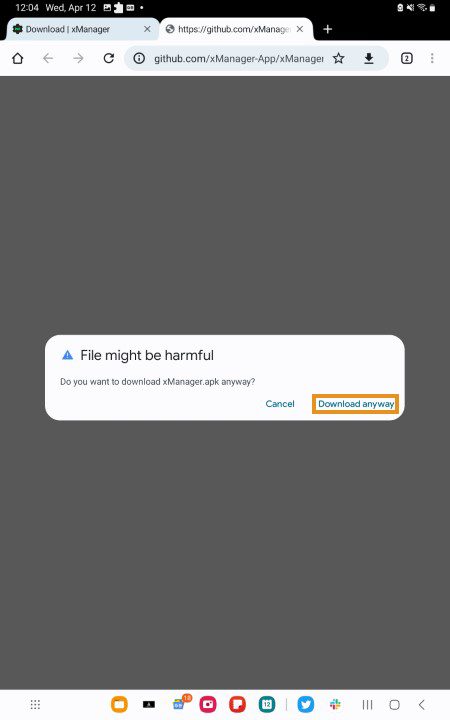In the image, the top section appears to be a screenshot from a mobile phone, exhibiting typical interface elements. The status bar is black, displaying the time: 12:04, in white. Beside the time, additional white text indicates the day and date as "WED, APR 12."

Below the status bar, there are two browser tabs visible. The first tab is highlighted in light blue, with the text "Download" in black and, vertically aligned next to it, "XSS Manager." The active tab is white with the URL "https://github.com/XMANAGE" truncated and ends with an 'X' for closing the tab, followed by a white plus sign (+) for adding a new tab.

Directly underneath the tabs is a gray toolbar. This includes a black home icon, two gray navigation arrows (one pointing left and the other right), a black circular refresh icon, and a gray oval containing a black circle with an 'i' (information) symbol within it. Adjacent to this, a text URL in black reads "github.com/XMANAGE-APP/XMANAGE," accompanied by a star icon and a download arrow.

Centered on the screen is a completely gray background with a white rectangular notification. Inside this rectangle, there is a blue triangle with a white exclamation mark, and the following warning message in black text: "File might be harmful. Do you want to download XMANAGER.APK anyway?" Two response options are provided: "Cancel," which is unhighlighted, and "Download anyway," highlighted in orange.